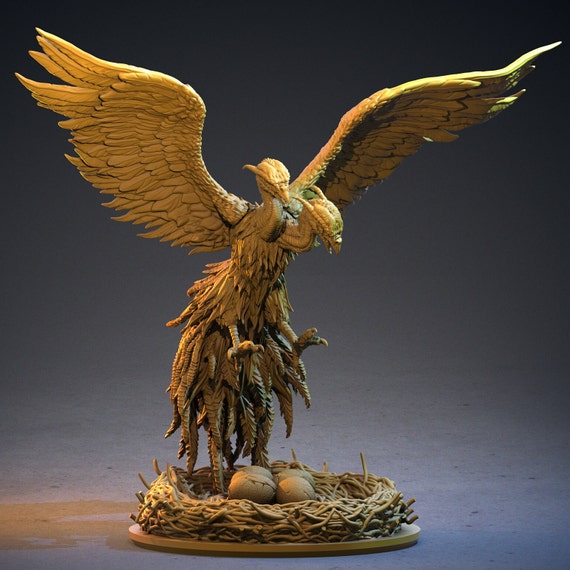This detailed image captures a golden-yellow statue with a slightly dark, ceramic-like finish intermingled with black textures, set against a dark gray to navy gradient backdrop. The scene is enveloped in a dramatic lighting effect, with a golden light illuminating the statue from the right upper corner, casting intricate shadows on the gray studio floor. The statue depicts a two-headed bird-like creature with expansive, detailed wings spread wide and webbed feet. The creature resides in an intricately designed nest, resembling intertwined spaghetti, which contains four slightly cracked, tan eggs. The bird’s feathers are meticulously textured, showcasing a blend of gold and black that emphasizes their lifelike appearance. The two heads, with beak-like structures and subtle horn-like protrusions, add to the mythical nature of the statue. The statue’s base and the nest are similarly colored, adding to the overall cohesive aesthetic of the sculpture. The complexity of the creature’s anatomy, including four clawed feet and a pair of prominent, widely spread wings, suggests a fantastical, almost dragon-like presentation. Despite the intricate design, the statue maintains a matte finish that contrasts with the shiny elements of the nest.